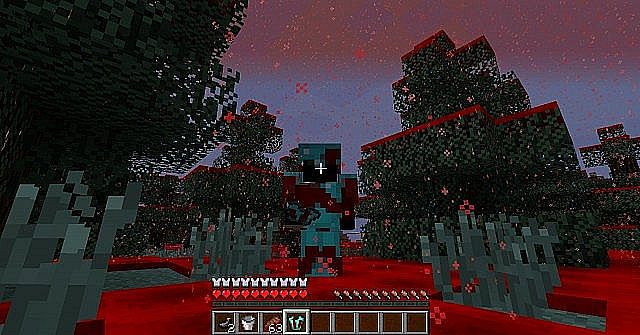A vibrant abstract image, with a predominance of green hues, appears to be a screenshot from a video game. The scene features several ambiguous structures, possibly resembling trees, standing against a dynamic backdrop of pinkish-blue sky. The base of the image is distinctly reddish, adding contrast to the overall green theme. At the bottom of the image, a series of selectable item boxes hint at its video game origin. The scene includes unique objects such as a cross-like figure and a centrally positioned, pinkish-colored star. A prominent green building with red stripes across its top adds intrigue to this slightly blurred yet captivating snapshot.